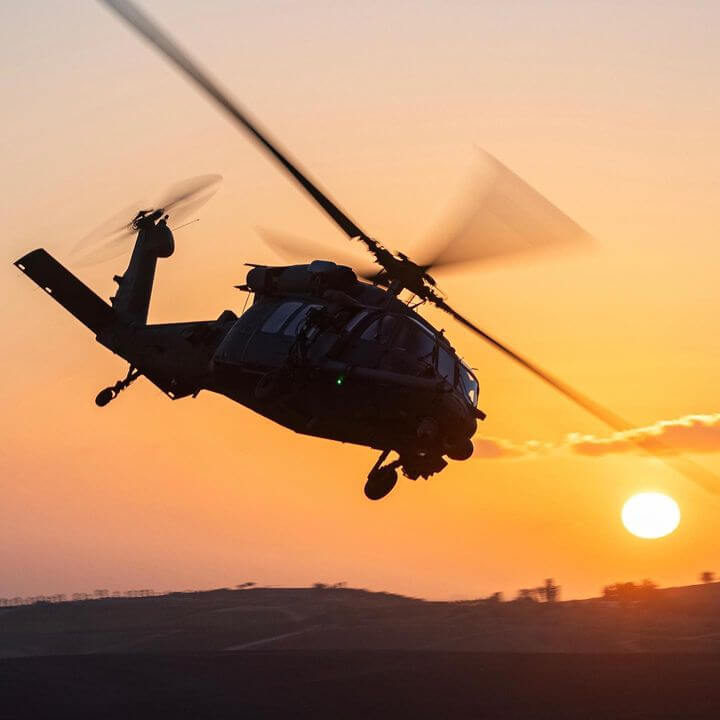This outdoor photograph, possibly a screenshot from a video given the noticeable macro blocking, captures a Pavehawk-type helicopter in mid-flight, angled toward the bottom right of the image. The helicopter’s black body is somewhat indistinct due to motion blur, especially noticeable in its rapidly whirring blades. Below the helicopter, a golden sun hovers just above the horizon, casting a brilliant, almost white glare that’s a trick of the eye. The sky is bathed in a gradient of bright orange near the horizon, transitioning to a softer peach higher up. Blurred background beneath the helicopter suggests the photo was taken while tracking its movement. Wispy clouds, tinged with the sun's orange glow, and a shadowy, tree-studded mountain range enhance the dramatic setting, indicating either sunrise or sunset.